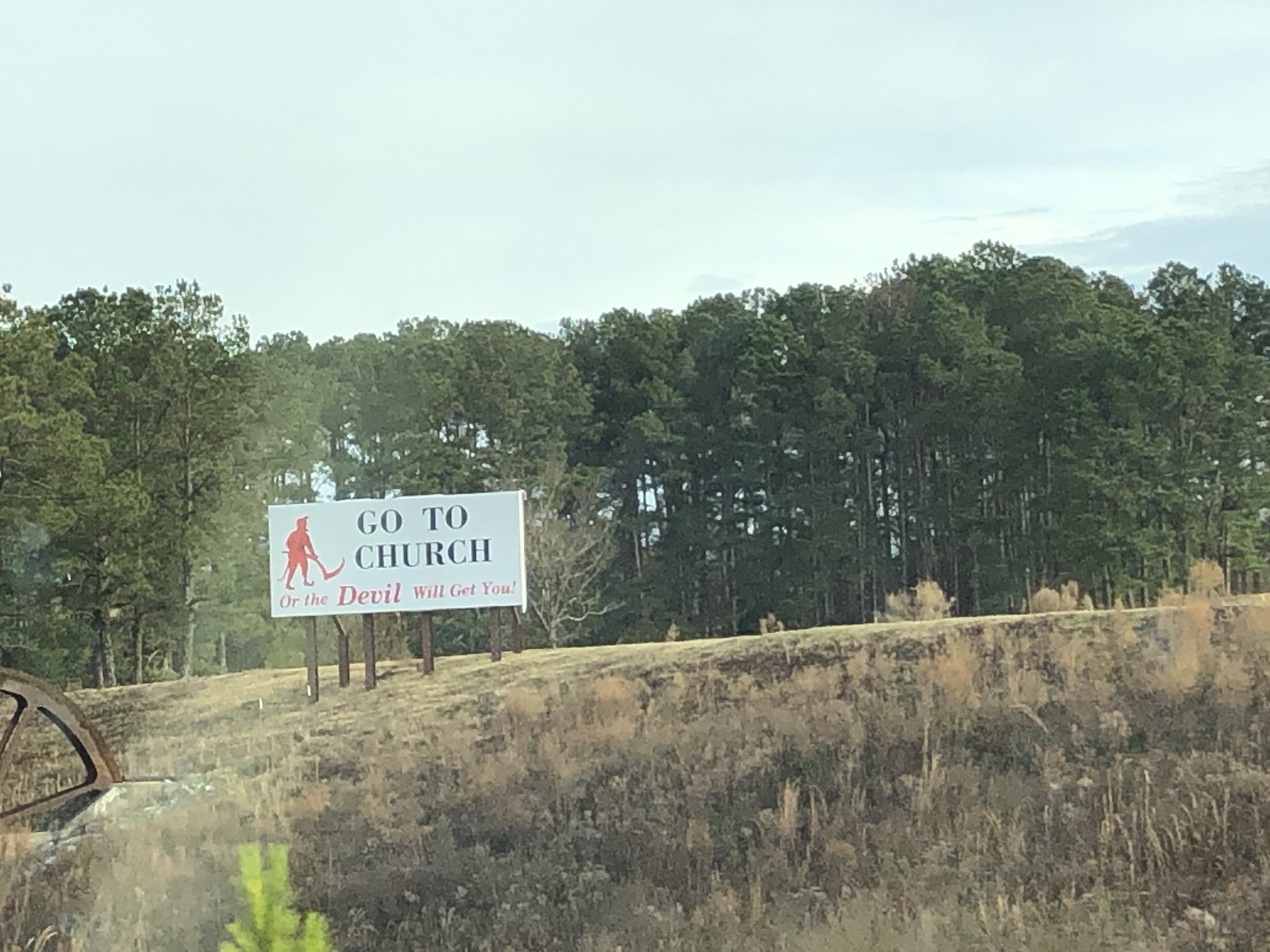The image prominently features a billboard with a stark, urgent message. At the top in bold, black, block capital letters, it reads "GO TO CHURCH." The words are split into two lines, with "GO TO" on the first line and "CHURCH" on the second. Below this, in striking red letters, the warning continues: "OR THE DEVIL WILL GET YOU!" followed by an exclamation point.

In the upper left corner of the billboard, there is an illustration of a devilish figure. This character has a long, pointed chin, and either sharp hair or a horn that tapers to a point at the forehead. The devil is holding what appears to be an agricultural tool resembling a scythe, typically used for cutting grass or tall plants. The figure also has a long, pointed tail and wears shoes with curling, upward-pointing toes.

To the left of the devil's image, there is a partial view of a large circle, likely part of a wheel, colored in brownish metal with patches of moss clinging to its surface.

In the foreground, the ground is covered with various grasses, predominantly in shades of brown and yellowish-green. A patch of greener grass is visible in the lower left corner. The landscape features a ridge that rises to the right and gently slopes down to the left, with tall trees dotting the horizon beyond the ridge.

The sky above is a gradient of light to darker blue, with fluffy clouds scattered across it, adding a sense of depth and open space to the scene.